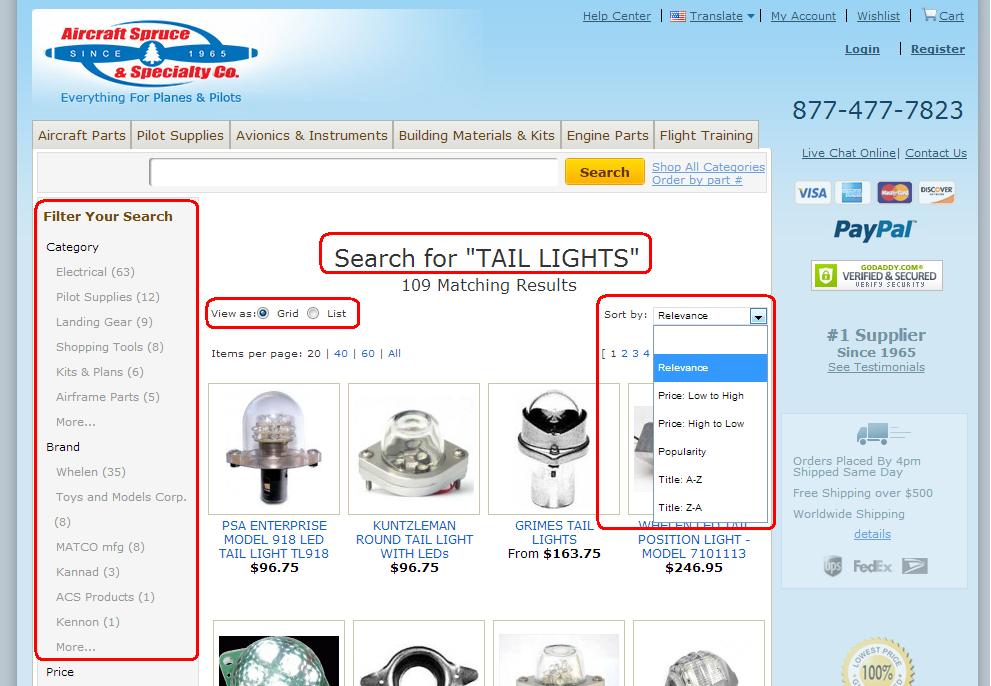A detailed image of a website titled "Aircraft Source and Specialty Co." The focus is a circular emblem featuring an airplane propeller with the inscription "Since 1965" in the center. At the top left, navigation tabs labeled "Help Center," "Translate," "My Account," "Wish List," and "Cart" are visible. Below these tabs, categories such as "Aircraft Parts," "Pilot Supplies," "Avionics," "Instruments," "Building Materials and Kits," "Engine Parts," and "Flight Training" are listed. Featured prominently on the page is a red-outlined box with a search field labeled "Filter Your Search," displaying the search term "taillights." The search results indicate "109 matching results," showcasing several types of devices related to the search query.